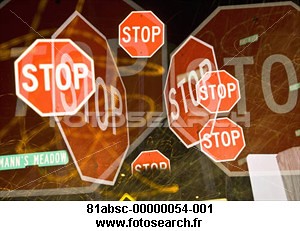This visually captivating graphic showcases a variety of American-style stop signs in assorted sizes and perspectives, creating an intricately layered composition. The image features four small, two medium, and three large stop signs, all overlaid atop each other at different angles and distances, imparting both vivid and transparent qualities to the signs. The classic red, white-bordered, octagonal signs are prominently displayed against a dark, nighttime backdrop that highlights strings of yellow light, adding a dynamic, almost laser-like effect to the scene. The lower left corner reveals a green street sign with white lettering, identifying the location as "Man's Meadow." At the bottom of the graphic is black text with the reference number "81ABSC-00000054-001" followed by the URL "www.photosearch.fr," suggesting the image is likely an artistic photograph taken from the inside of a shop window. The reflective quality of the glass creates an illusion of more signs, emphasizing the multiple layers and giving the impression that the shop specializes in selling these iconic roadside symbols.